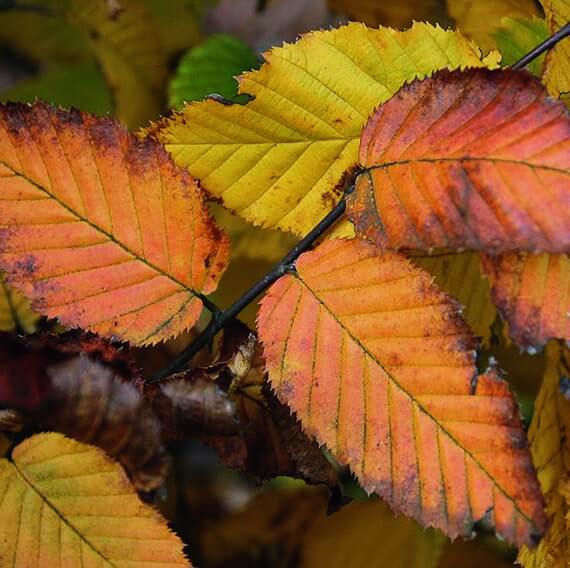This close-up color photograph showcases a vivid array of autumn leaves, primarily in orange and yellow hues, with some displaying rich, pumpkin-like orange and lemon-yellow tones. The leaves, teardrop-shaped with frayed, jagged edges, convey the varied stages of their fall transformation, from vibrant shades to darker, brown-tinted edges where they are beginning to dry and decay. A thin, brown tree branch is visible, connecting several leaves in the foreground, where up to five leaves are distinctly seen. In the background, which is somewhat blurred, a mix of green leaves, likely lime green, and a few completely dead, dark brown leaves can be discerned, painting a complete picture of the tree's foliage in different phases of autumn. The intricate veins of the leaves are apparent, adding to their detailed texture, reminiscent of the season's natural beauty.